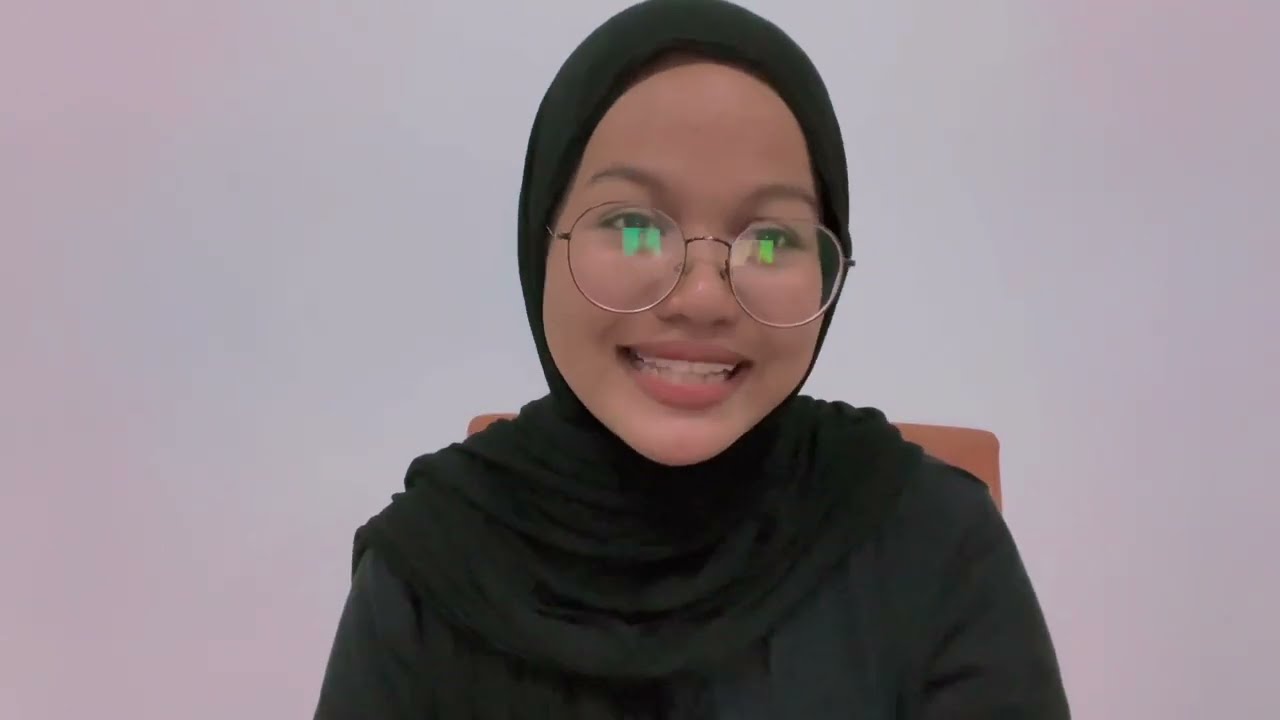This photograph depicts a woman, wearing a full black hijab and matching long-sleeved garment, seated comfortably on a brown, wooden chair. The background is a plain grayish-white wall with a slight pinkish tint. The woman, who appears to have an olive tan complexion, is smiling warmly, her large, round glasses reflecting a hint of green light, possibly from a screen in front of her. Her black hijab, made of a thick material, fully covers her hair and wraps around her head and down her torso, giving a scarf-like effect around her neck. She is the sole subject of the image, with no other people, objects, or text present. The top of her head is slightly cut off in the frame, emphasizing her joyful expression and modest attire.